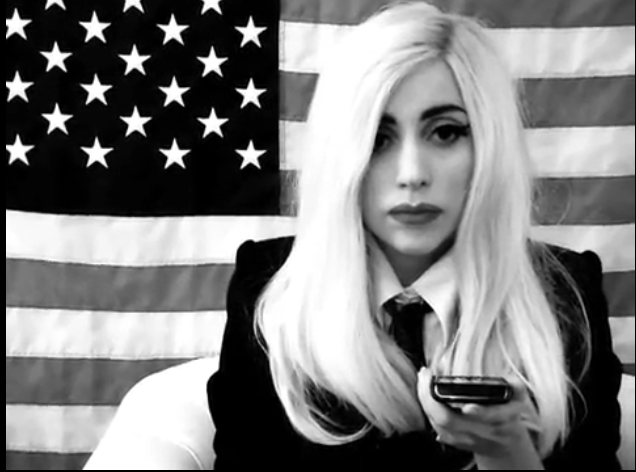This striking black-and-white photograph presents a poised woman with a contemporary style. The subject is a blonde woman dressed in a tailored suit, featuring a black coat layered over a crisp white dress shirt, accentuated with a sleek black tie. Her hair, although blonde, appears almost white due to the monochromatic filter, with contrasting black roots suggestively peeking through where her hair parts to the left. She sports thick black eyebrows, dense black eyelashes, and full oval lips that lend a dramatic flair to her face.

Sitting elegantly on a white faux leather couch, she holds what seems to be either a remote control or a smartphone in her left hand. Her gaze is directed off-camera, adding a layer of intrigue to the composition. The backdrop draped with an American flag spans the entire wall, creating a bold and patriotic aesthetic. Her hair falls straight and is meticulously parted to her left side, framing her face perfectly.

The photograph exudes a photoshoot atmosphere, meticulously crafted to highlight the subject's sophisticated and edgy demeanor.